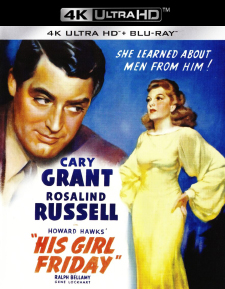The image depicts a slip cover for a 4K Ultra HD Blu-ray disc of the classic movie "His Girl Friday," featuring Cary Grant and Rosalind Russell. At the very top, the label reads "4K Ultra HD" in white text on a black rectangle, with "4K Ultra HD Blu-ray" printed below on a gray label. The movie's title, "His Girl Friday," is prominently displayed in red at the bottom. The cover includes a tagline in white capital letters, "She Learned About Men From Him!" against a blue background. Cary Grant's name appears in blue, followed by Rosalind Russell's, and then Howard Hawks in smaller blue text. Ralph Bellamy's name is also listed in blue. The upper left displays an image of a man with short black hair in a red suit, likely Cary Grant, while the right side showcases a woman, likely Rosalind Russell, in a yellow gown with red hair, both hands on her hips. The lower right corner of the cover is depicted in black, adding a touch of contrast. This cover art emphasizes the 4K Ultra HD quality and the film's vintage charm.